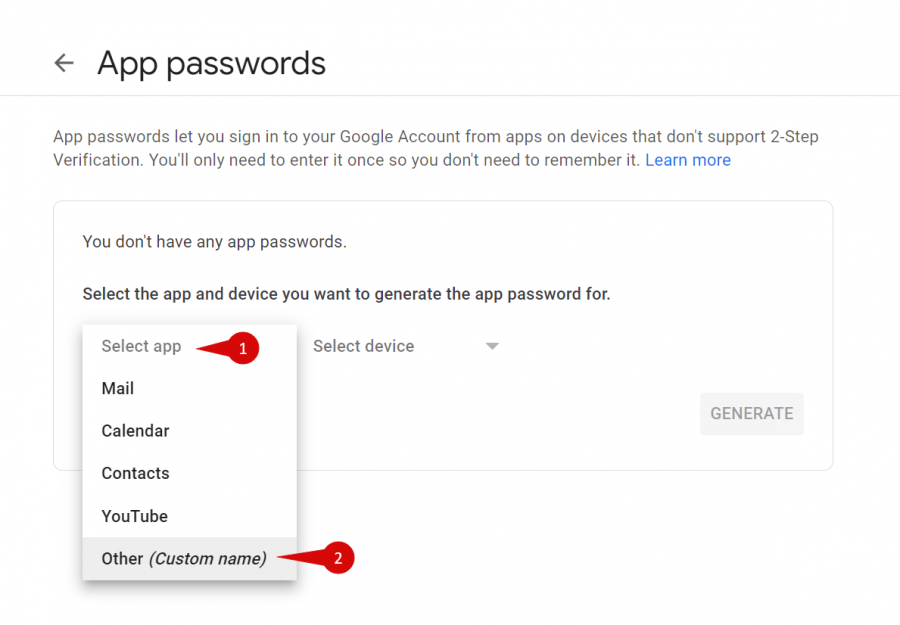**Detailed Caption:**

A screenshot of a "App Passwords" page related to Google account security. The top of the image features the heading "App Passwords" in black text, accompanied by a back arrow icon. Just below the heading, a descriptive text in black reads: "App passwords let you sign into your Google account from apps and devices that don't support two-step verification. You only need to enter it once so you don't need to remember it." Adjacent to this statement, a "Learn more" link in blue is available for further information.

Beneath this section, there is a notification stating, "You don't have any app passwords." Following this text, an instruction in bold highlights: "Select the app and device you want to generate the app password for." Under this directive, within a red circle marked with a white number "1" and an arrow pointing towards it, the option "Select app" is shown.

Below the mentioned red circle, a list in bold offers options such as "Mail," "Calendar," "Contacts," "YouTube," and "Other (custom name)." The text "Other (custom name)" is displayed in gray. Beside this list, another red circle marked with a white number "2" includes an arrow pointing to the options.

Overall, the image gives comprehensive instructions and illustrations on generating app passwords for use with various applications and devices that do not support two-step verification.